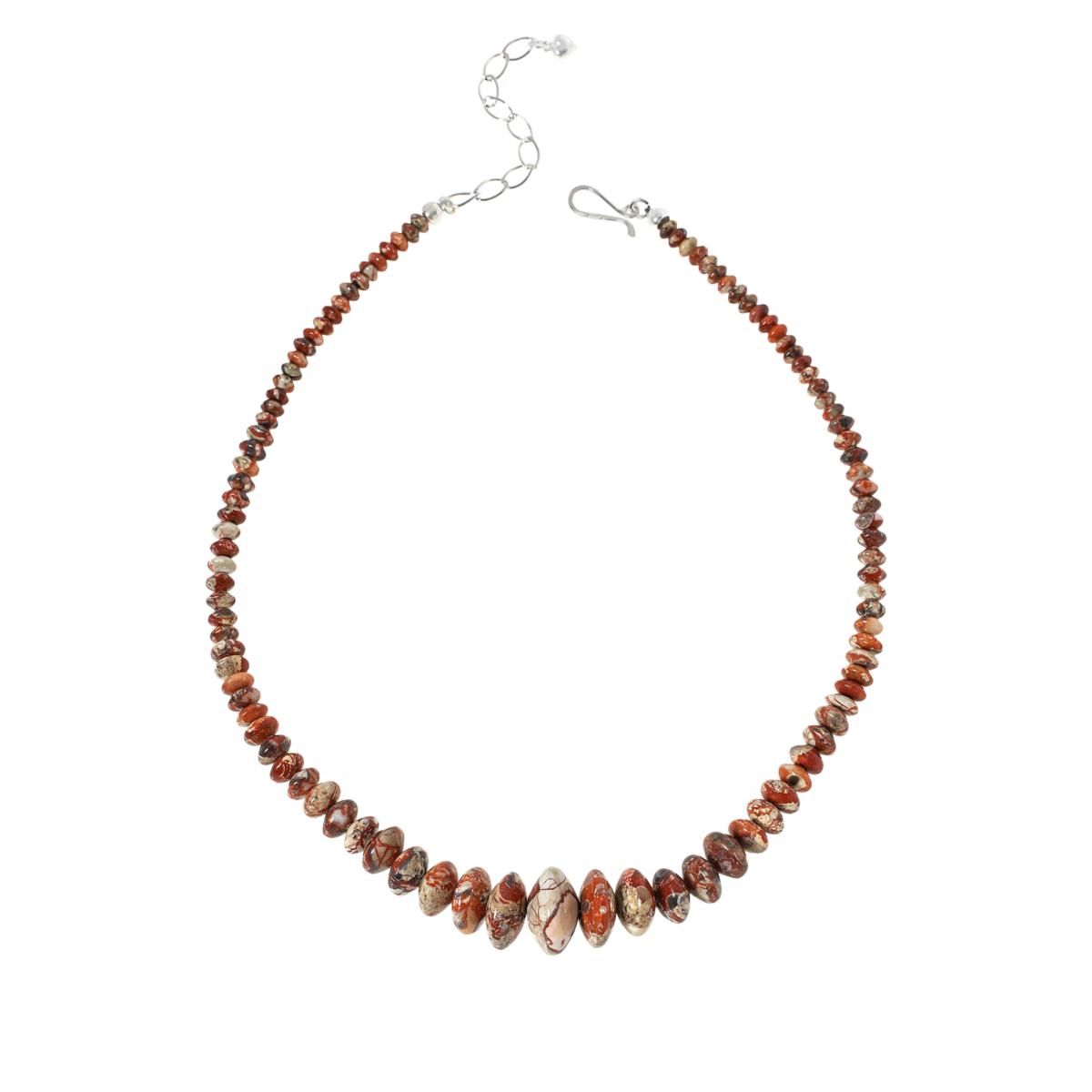The photograph captures a beautifully crafted stone necklace displayed against a pristine white background, enhancing its vibrant colors. The necklace, photographed in a portrait orientation, features a series of graduated stones, increasing in size towards the largest central stone. This centerpiece stone is predominantly white and gray with hints of brown and a striking red line crossing through it, accompanied by a small red section at the top left. The surrounding stones display a captivating marbleized effect with variegated colors, including cream, rust, light green, brown, and subtle orange hues, all polished to a smooth finish. The necklace is arranged in a circular shape, lying flat with a delicate silver clasp on the top right and an adjustable chain with multiple links ending in a small silver ball on the top left. The conical, slightly flattened stones give the piece a modern yet timeless aesthetic, all while the necklace appears to float gracefully on the white backdrop, embodying photographic representationalism realism.